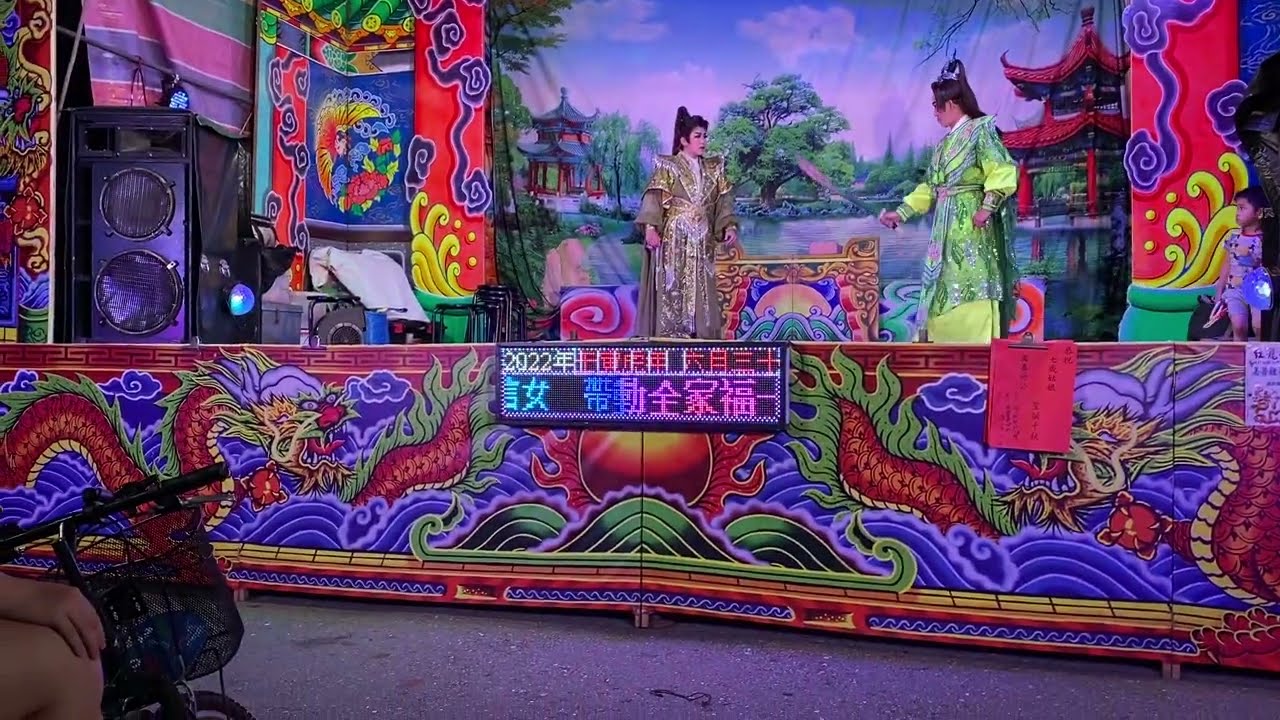This highly detailed photograph captures a vibrant and elaborate stage scene from an Asian opera or play. The stage is adorned with a vividly painted backdrop featuring a serene lake, lush green trees, and a traditional pagoda, all framed by elegant red curtains on either side. Two actors, both with long hair and dressed in flowing, ornate robes, stand facing each other. The actor on the right, clad in a richly decorated green and gold robe, appears to be holding a sword in his right hand. Opposite, the actor on the left wears a luxurious silver robe, his hands empty. The stage's front facade is equally ornate, showcasing intricate dragon figures in purple, orange, and green hues. At its center, a panel displays text in Asian characters.

Adding to the scene's complexity, a person's hand and leg, along with a bicycle's front wheel and basket, are visible at the bottom left corner, suggesting the presence of a mural on a city street. Additionally, a large black speaker is situated on the left of the stage, while another figure appears to be watching from behind the scenes on the right. The ground beneath the stage is gray asphalt, further hinting at an outdoor, mural-like setting. Overall, the image bursts with color and detail, merging theatrical elements with urban life.